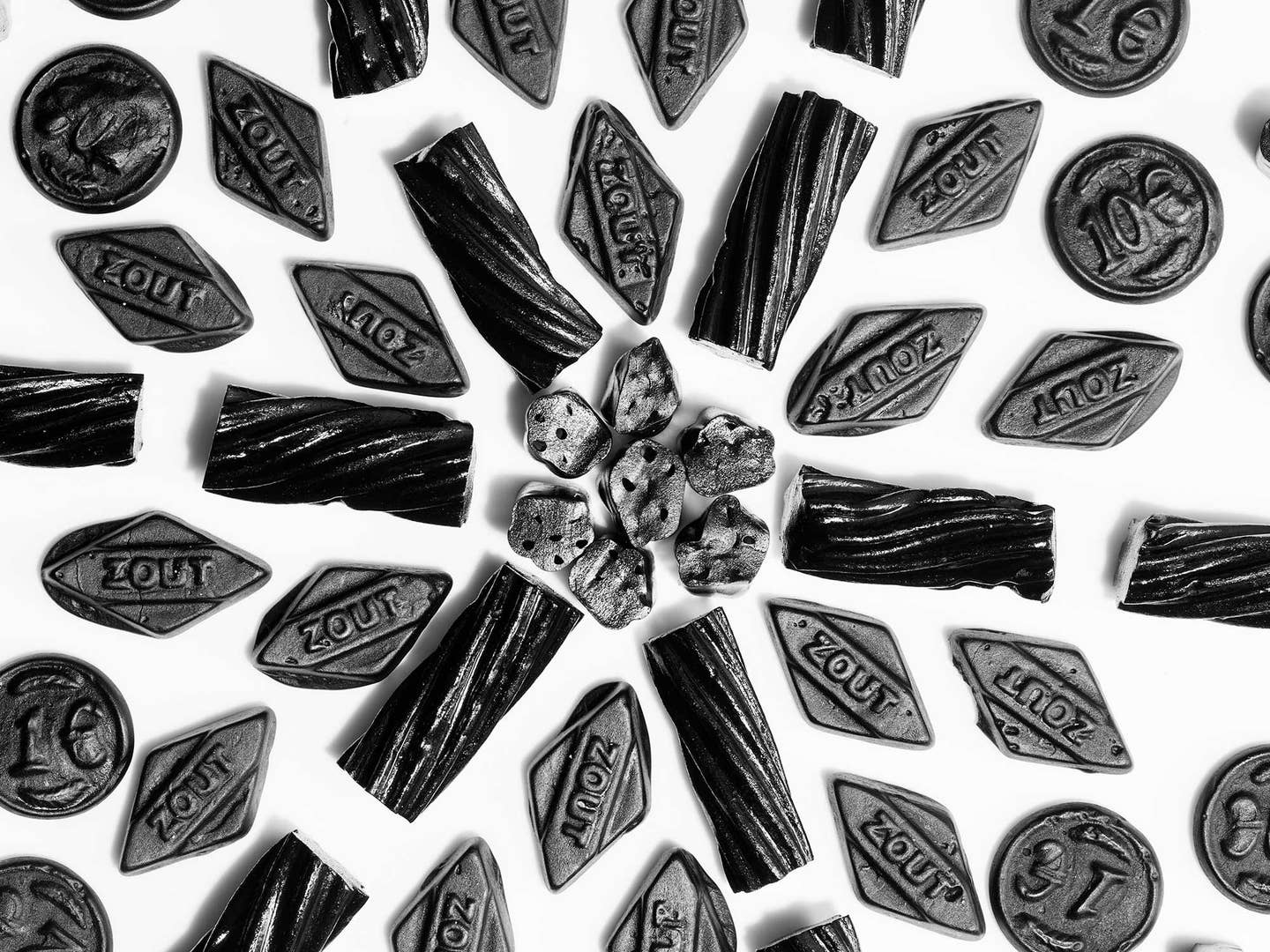This is a black and white photograph displaying an intricate artistic arrangement of various types of black licorice candy on a crisp white background. At the center, six chocolate chip-like candies form a circle, radiating outwards with six twisted licorice pieces. These spirals create a starburst effect, interspersed with diamond-shaped licorice candies inscribed with the word "Zout." Surrounding these are round coin-shaped candies, some labeled with "10 Euro," "1 Euro," or featuring animals. The pattern continues outward, maintaining a detailed, flower-like design, with the coins filling in the gaps and enhancing the overall composition. This captures not just a confectionery delight but also an exemplary display of candy arranged with precision and aesthetic consideration.